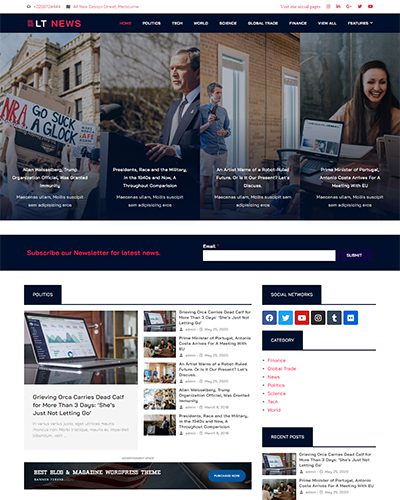This image is a screen capture of a news website featuring a clean, white background with dark blue banners and section headings accentuated by white text, along with sporadic splashes of blue and red text. While much of the smaller text is unreadable, the top of the page prominently features a white section with several red social media icons, indicating links to platforms such as LinkedIn, Twitter, and YouTube. Below this line, a blue banner displays a small logo followed by the letters "LT" in bold white block letters, and the word "News" in bold red block letters. 

Adjacent to the logo is a navigation bar, with the first tab labeled "Home" in red, while the subsequent tabs including “Politics,” “Tech” (potentially), “World,” “Science,” “Global Peace” (or a similar phrase), “Finance,” “View All,” and "Features," are in white font. The "Features" tab also includes a small drop-down icon next to it.

Below this navigation bar, the page segments into several photographs, the most prominent of which features former President George W. Bush standing at a podium delivering a speech.